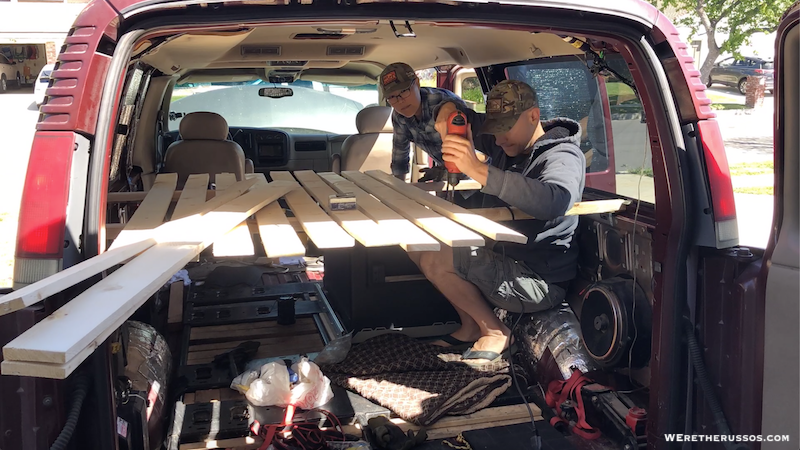In this detailed photograph, two men are seen working inside the back of a maroon-colored van, with all its doors wide open. The men, both white and wearing camouflage baseball caps, are engaged in a woodworking project. The man on the right, who is seated on a rolled-up rug or insulation, is holding a drill and wearing flip-flops along with a jacket with a hood and shorts. He is focused on drilling a vertical plywood slat into a horizontal one, possibly assembling a shelving unit or a makeshift table in the van. The man on the left, who is older and wearing a blue and white checkered shirt with glasses, observes the drilling process.

The van's interior is cluttered with various items, including plastic bags, two by fours, wires, and rolled-up materials that resemble moving van wrappers. The background suggests they are in a residential neighborhood, as driveways and cars are visible, along with trees and a fire hydrant on the right side. Notably, the bottom right corner of the image bears the text "We're the Russos dot com."